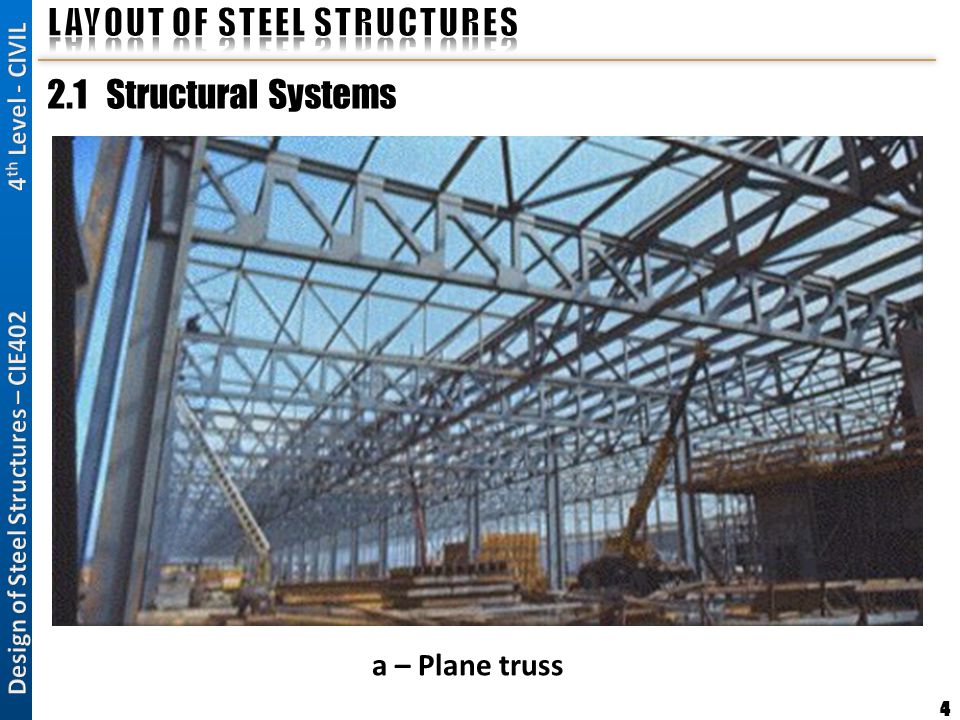The image depicts a partially constructed large steel truss structure, possibly the framework of an aircraft manufacturing facility or a large warehouse. The spacious area beneath the truss is filled with cranes and various construction materials scattered on the ground. The structure lacks a roof, allowing the sky to be visible. The slide, which appears to be part of a presentation or educational material, is titled "Layout of Steel Structures." Below this heading, it reads "2.1 Structural Systems." A vertical blue ribbon on the left side of the slide features the text "Design of Steel Structures, CIE 402, 4th Level - Civil." The slide number "4" is located in the lower right corner. The main image is primarily composed of blue, gray, brown, tan, black, and white colors, emphasizing the industrial and work-focused environment of the scene.